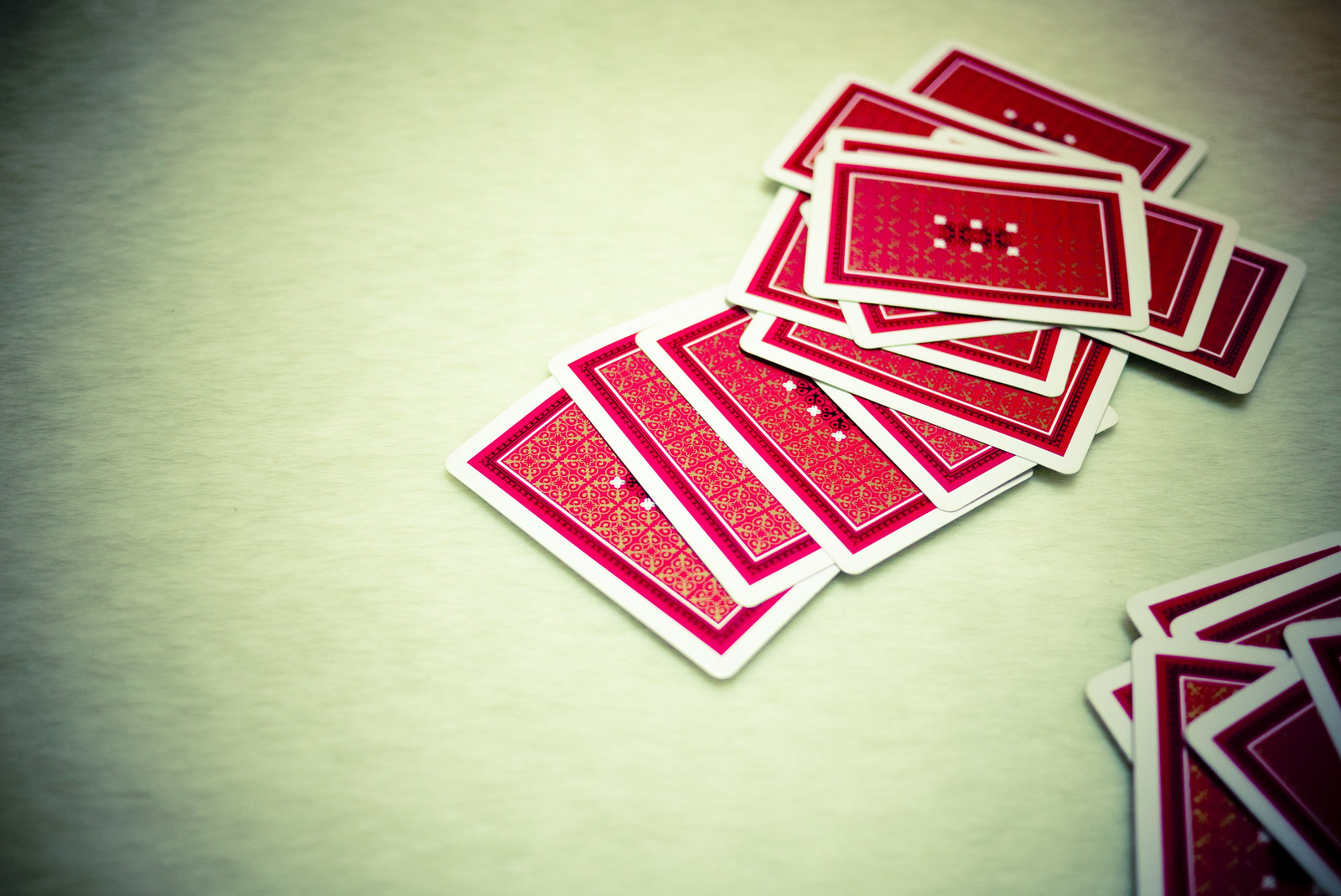This is a close-up photograph of a table set for a card game, captured in a rectangular, landscape view. The table features a light yellow surface that contrasts beautifully with the dark gray and black shadows framing the left and right sides of the image. Scattered across the table are playing cards, characterized by a striking design: each card has a white border surrounding a dark red rectangle, which encloses a smaller white rectangle at its center. Intricately placed within these white rectangles are small designs composed of black lines and white dots. A number of cards are arranged in a cascading manner from the top right corner to the center of the image, while another substantial stack of cards rests in the bottom right corner.